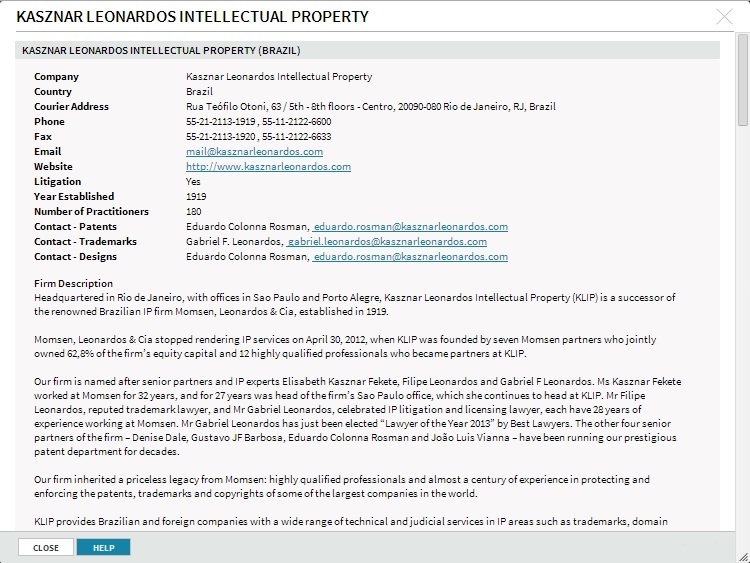"**Casanare Leonardo's Intellectual Property**: This detailed informational website provides comprehensive insights into Casanare Leonardo's Intellectual Property (KLIP), a prestigious Brazilian firm specializing in Intellectual Property services. Founded in 1919, the firm has established itself as a leader in the IP sector, with its principal office in Rio de Janeiro and additional offices in São Paulo and Porto Alegre. 

KLIP is the successor to the esteemed Brazilian IP firm, Momsin, Leonardo's and SIA, which ceased providing IP services on April 30, 2012. The transition to KLIP was led by seven Momsin partners, collectively owning 62.8% of the firm's equity capital, alongside 12 distinguished professionals who also became partners.

Key contacts at KLIP include Eduardo Colonna Rosman for patents and designs, and Gabrielle F. Leonardo's for trademarks. The firm boasts a robust team of 180 practitioners and has been instrumental in various IP litigations. The website provides essential information including the firm's contact details (phone, fax, email), although the courier address is in Portuguese.

With its long-standing history and a team of highly qualified professionals, KLIP continues to uphold its legacy of excellence in the IP domain."